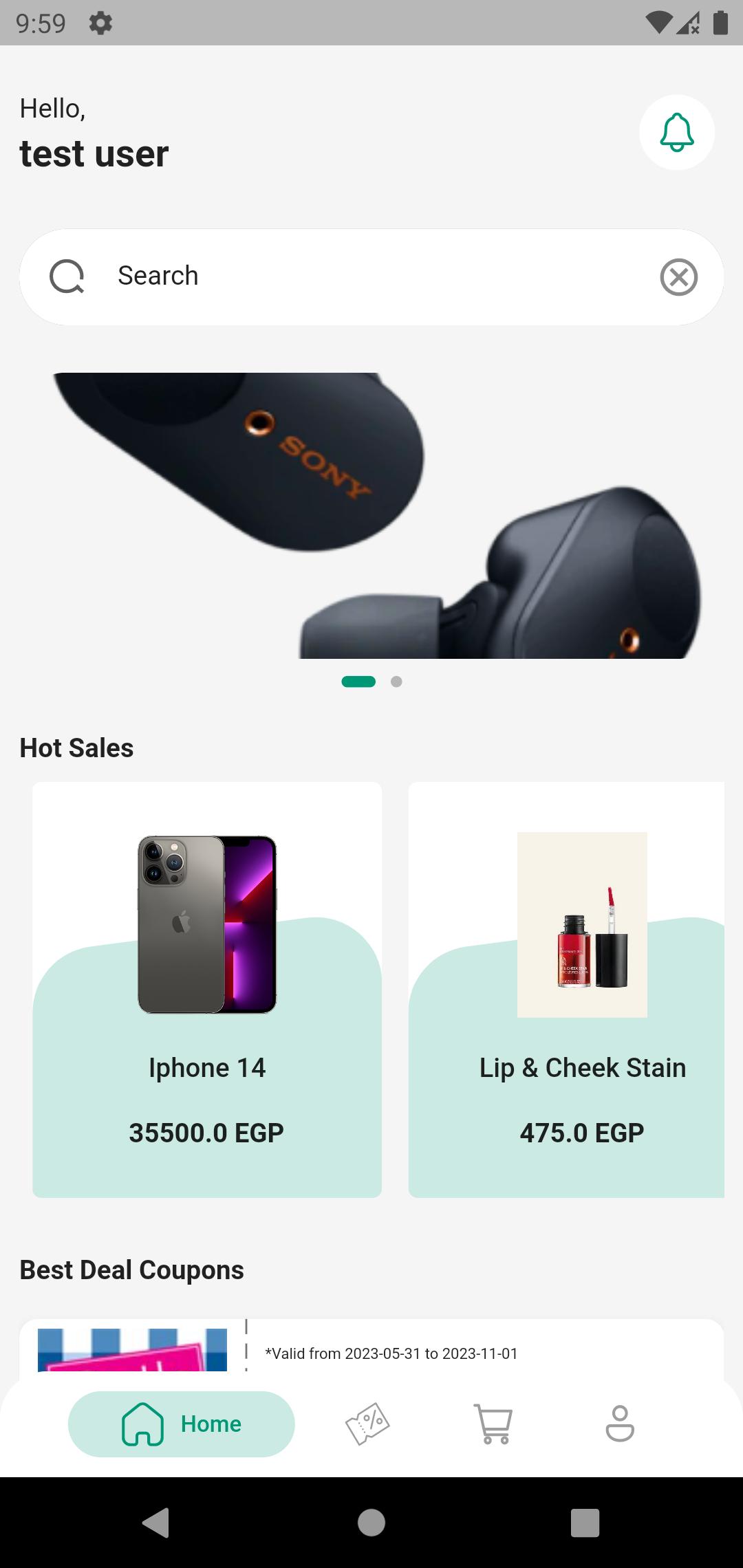The image is a screenshot of a smartphone screen displaying an interface at 11:59 AM. In the upper left-hand corner, the time is indicated next to a settings icon. The battery life indicator shows a full charge. Below the time, there is a greeting message, "Hello test user," where "Hello" is in a smaller, plain font, and "test user" is in bold, lowercase letters. A green notification bell icon is situated to the right of the greeting.

Directly beneath the greeting, there is a search bar with options to search or exit. Below the search bar, there is an image of a unique type of speaker by Sony, featuring a central hole that appears to accommodate a screw, possibly for mounting or setup purposes.

Further down, the interface displays a section titled "Hot Sales." On the left, it showcases an iPhone 14 priced at 35,500 EGP (Egyptian Pounds). To the right, there is an advertisement for a "Lip and Cheek Stain," effectively a type of lipstick or cosmetic paint, priced at 475 EGP. Additionally, there is a mention of "Best Deal Coupons Available," with a clickable link to explore coupon details. These deals are valid from May 31, 2023, to November 1, 2023.